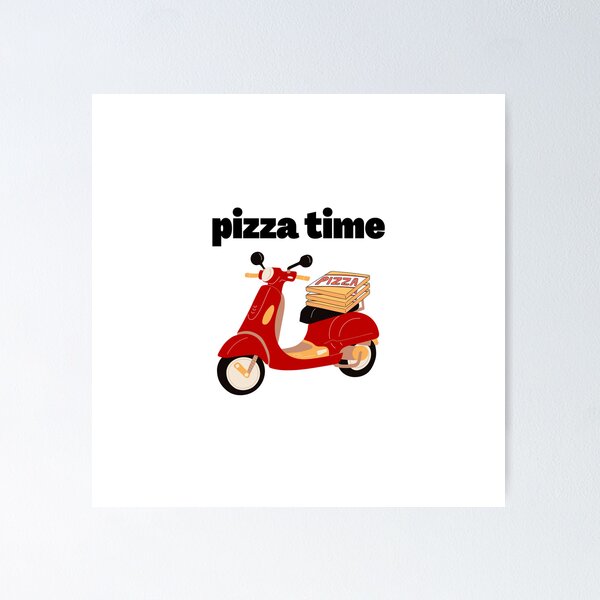The image features a white square poster centered on a large light grey frame-like background. At the heart of the poster is a stylized, red Vespa-like scooter with beige trim, black tires with whitish-gray rims, black mirrors, and yellow handlebar ends. The scooter, which faces to the left, is topped with a black seat holding three yellow pizza boxes labeled "PIZZA" in red with a white line running through the design. Above the scooter, in bold black font, the phrase "pizza time" is prominently displayed in lowercase letters. The overall scene captures a vibrant and minimalistic depiction of pizza delivery.